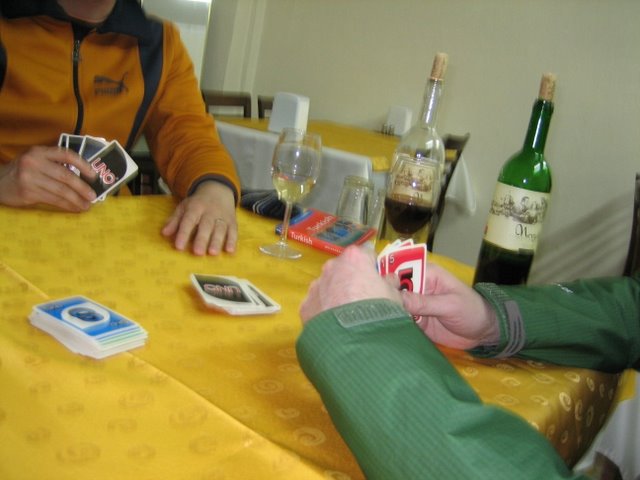In this captivating image, two individuals are engrossed in a lively game of Uno, seated at a table draped with a tablecloth. On the table, you can spot a vibrant deck of Uno cards, suggesting a fun-filled game night. Beside them, there are a couple of wine bottles and a wine glass that is approximately one-third to one-half full, indicating a relaxed and convivial atmosphere. Adding an intellectual touch, a book on learning the Turkish language rests on the table, hinting at a possible interest in travel or language acquisition.

The person on the left is clad in a distinctive green jacket adorned with gray clasps at the cuffs, while the person on the right sports a rust-colored jacket featuring a black collar and black trim. These players, who could be of Caucasian, Hispanic, or Asian descent based on their skin tones, show a diverse gathering of friends.

In the background, a yellow table accompanied by three chairs can be seen, suggesting that the setting might be a cozy restaurant perfect for social gatherings and game nights.